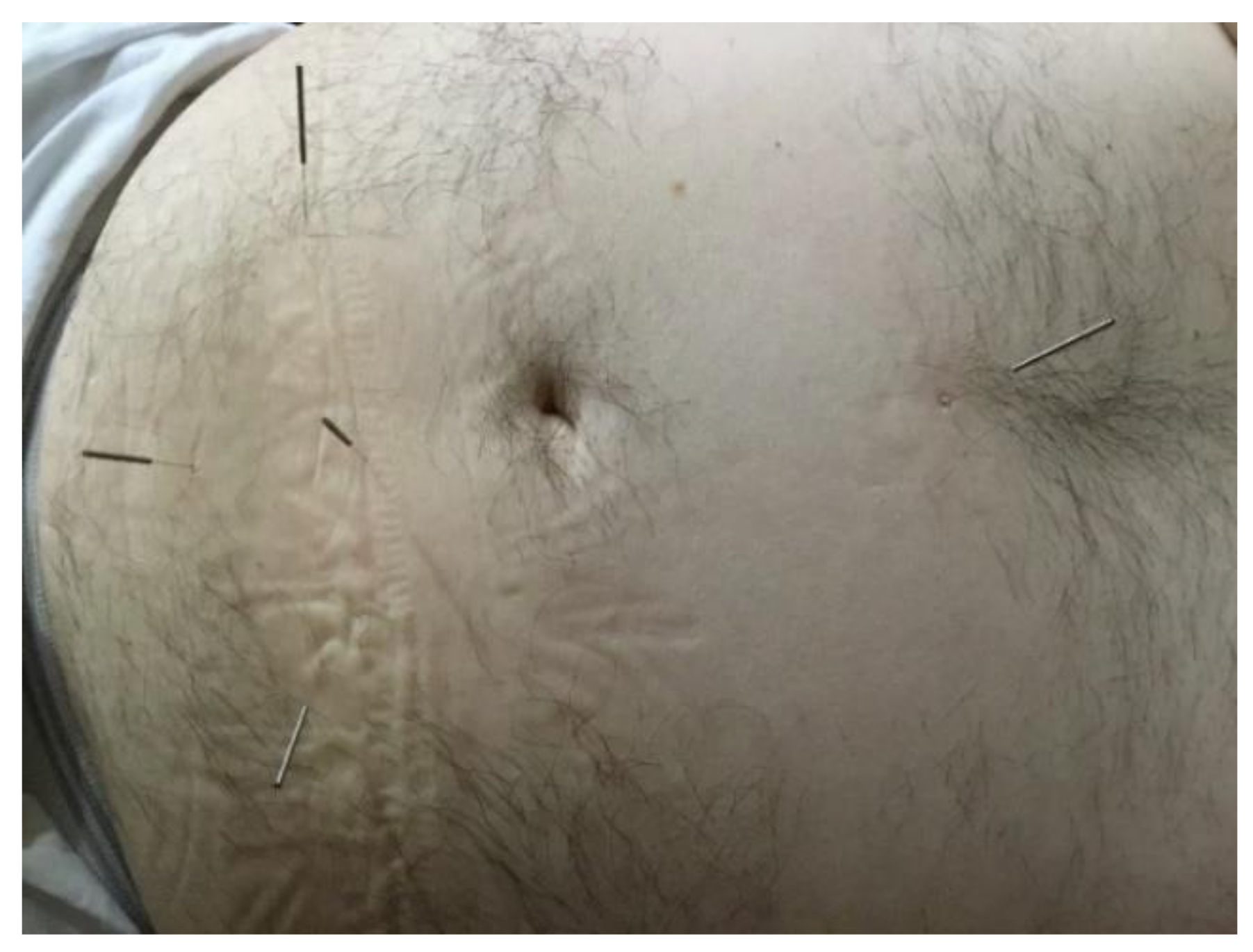The image depicts a pale, hairy male abdomen, prominently displaying a belly button. The stomach, which occupies the entire frame, appears slightly wrinkled, suggesting some age or a relaxed state. Five acupuncture needles can be seen puncturing the skin; four of these needles are close together below the navel in the lower middle and lateral regions, with one positioned above the navel. The needles appear black. There is a bit of a white t-shirt visible in the upper left corner and a slight towel draped on the left side of the image, lending a clinical or therapeutic setting to the scene.